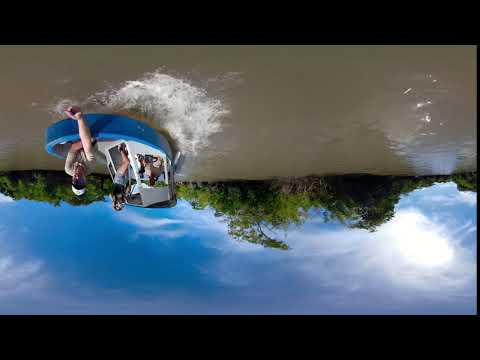An upside-down photograph depicts a group of three people in a blue and white watercraft on a body of light brown, murky water that appears at the top due to the orientation of the image. White water sprays off the side of the floating raft they are on. One man in the boat is wearing a white hat and a light gray short-sleeved shirt, while another person beside him is dressed in a black shirt and blue shorts. Behind them, there is a thick line of dense green trees, with one tree notably pointing to the right and another forming a distinctive bump. The background unveils a sky—mostly blue on the left side—transitioning to a swirl of white clouds on the right, where a bright light shines through. The image is framed with black borders at the top and bottom, emphasizing the outdoor setting under daylight, captured from the perspective of another boat.